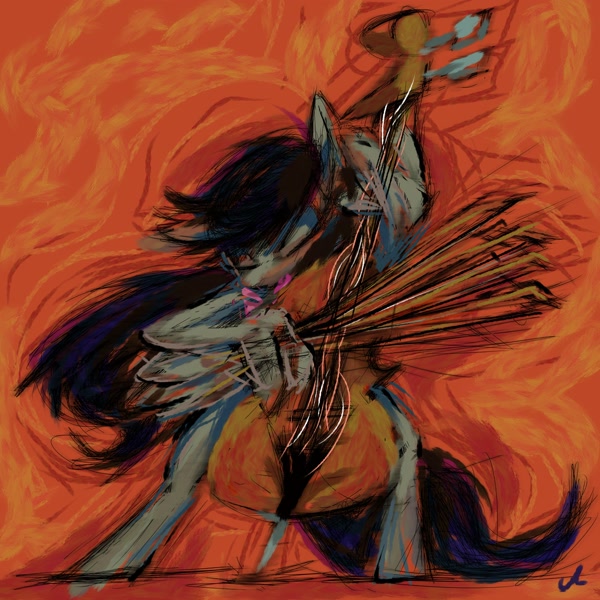The artwork depicts an enigmatic figure, possibly an anthropomorphic creature with long, flowing black hair and pointy ears, reminiscent of a mythical animal such as a horse or unicorn, fervently playing a cello. The figure's dynamic motion is captured with the bow in hand, suggesting vigorous, fast-paced playing. The sweeping illustration is rich in color, dominated by fiery hues of orange and red that intensify towards the center, creating an almost flame-like background. The cellist's instrument is depicted in shades of brown with black and gray accents, while hints of blue and purple add depth to the scene and highlight the figure's hair and surrounding environment. A signature, resembling the letter 'A,' is located in the lower right-hand corner, marking the artwork’s creator. The entire scene is bathed in vibrant colors and intense motion, emphasizing a dramatic and action-packed moment.